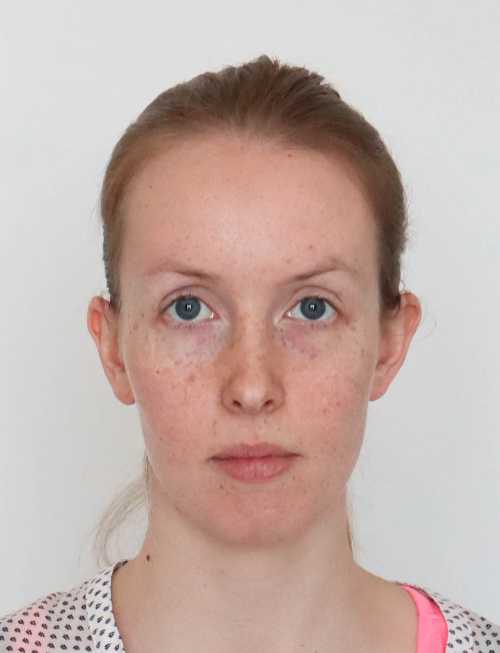The photograph features a close-up view of a young Caucasian woman, approximately 19 to 20 years old, standing against a solid white background. Her oval-shaped face is framed by red hair pulled back into a ponytail, leaving her forehead exposed and a small wisp draping down to her shoulder. She has blue eyes, complemented by sparse eyebrows that match her hair color. Her face, including her cheeks and nose, is lightly freckled. She appears to have no makeup on, presenting a natural look with closed lips and a neutral expression, resembling a passport or ID photo. She is clad in a white shirt adorned with black polka dots over a pink tank top, and her neck is bare save for a small mole on the right side. The overall composition conveys a straightforward, unembellished portrayal of the woman.